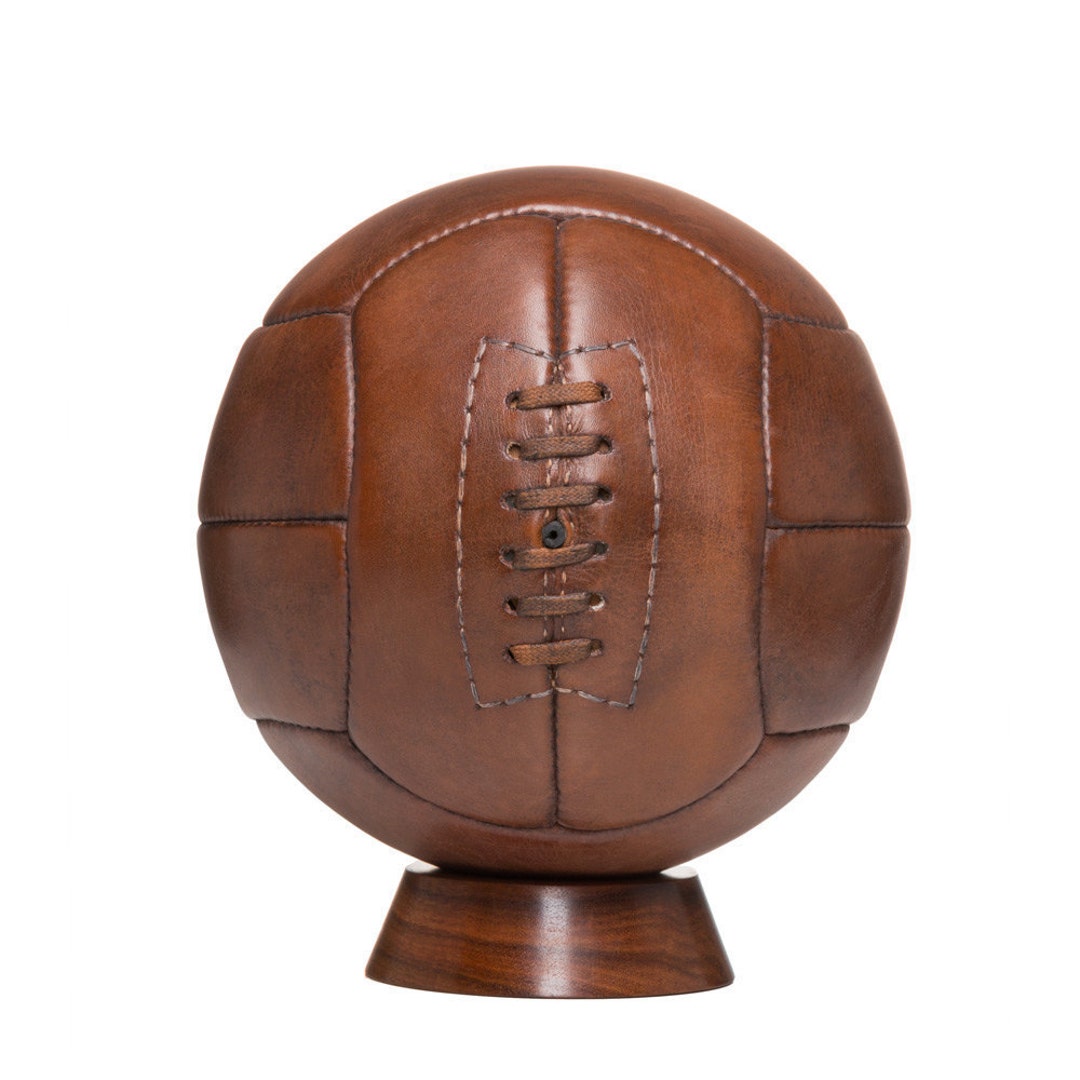This photograph showcases a vintage, early style football or soccer ball, commonly referred to as a football in European countries. The ball is crafted from brown leather, assembled in a patchwork design with multiple stitched panels. Prominent leather laces run across its center, tightening six lace points that hold the ball together. An air nozzle for inflating the internal bladder is located prominently in the middle of the ball. The well-oiled, glossy leather indicates careful maintenance and preservation over the years. The ball, measuring approximately 5 inches in diameter, is displayed on a polished, circular wooden stand, enhancing its antique appearance. The detailed craftsmanship of the stitching and the overall condition suggests it is a cherished vintage piece.